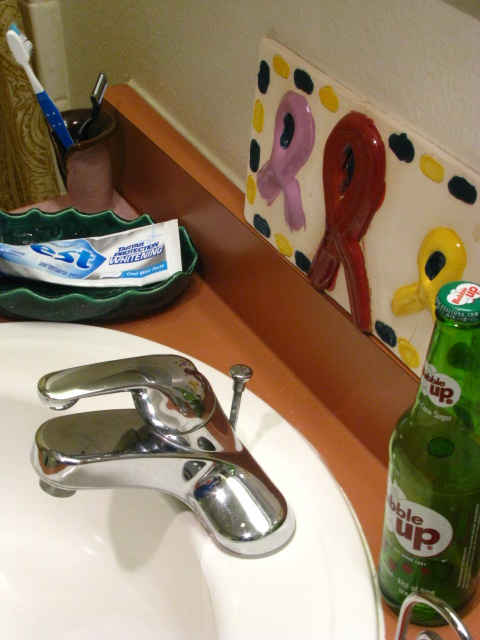The image depicts a personal bathroom countertop, providing an intimate glimpse into someone's private space. Dominating the scene is a tube of Crest Sensitive Protection Teeth Whitening toothpaste, perched on a uniquely wavy, greenish stand. Nearby, a glass can of Bubble Up juice, its brand name prominently displayed, adds a touch of refreshment to the setting.

The perspective of the image places us just above the sink, offering a partial view of the countertop and one edge of the sink basin. The sink's material appears somewhat cheap—possibly a faux wood—with a light orange-tan hue that gives off an earthy tone. The faucet, a single-hole fixture, is clearly visible, though the bowl of the sink remains mostly out of sight.

In the corner of the image, a purple cup holds several toothbrushes and a razor, indicating daily routines and personal hygiene habits. The cup features a design with ribbons reminiscent of cancer awareness symbols, adorned with navy yellow circles and intricate patterns of pink, red, and yellow ribbons. These small, yet significant, details provide a deeper layer of personality and lived experience to this everyday space.